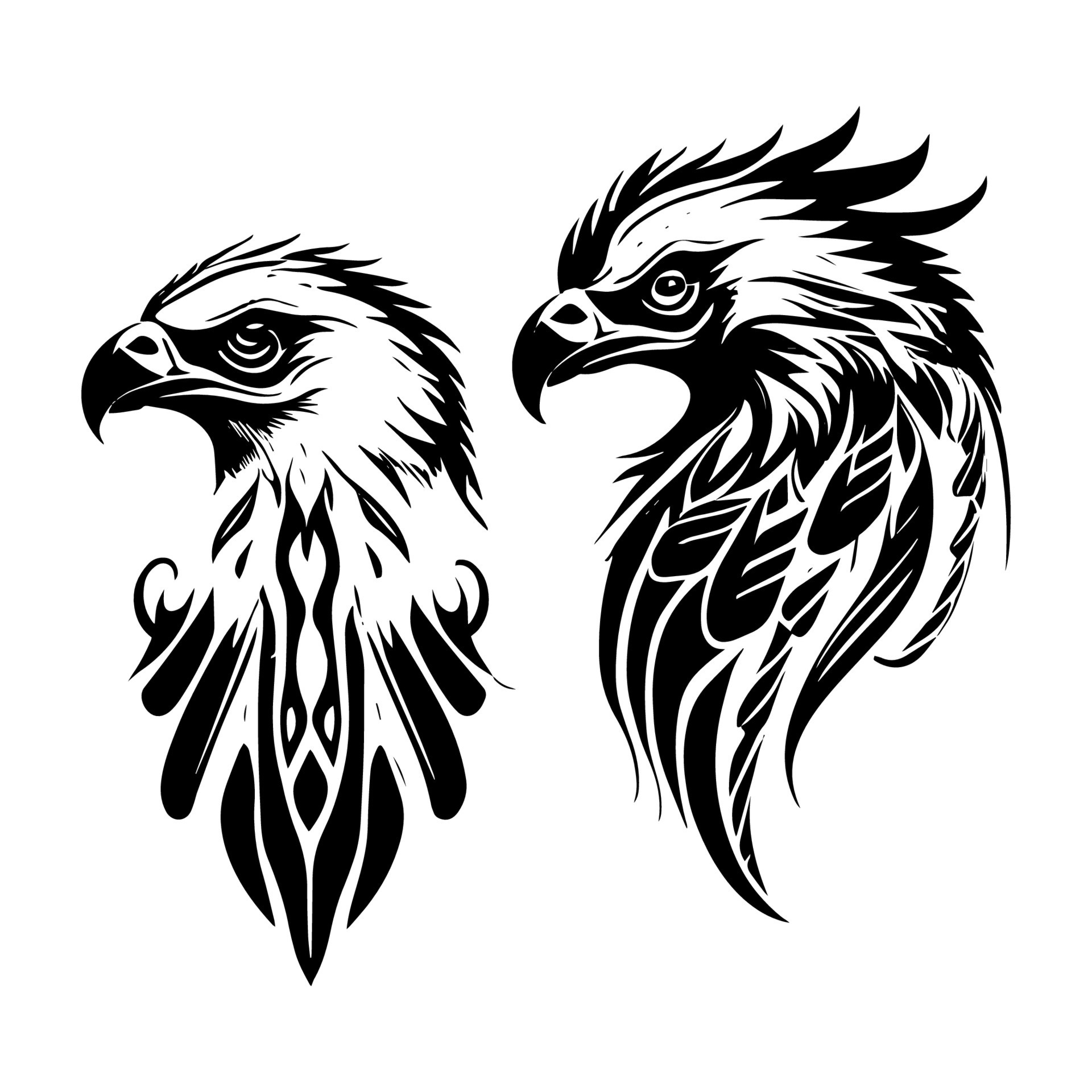In this intricate black and white line drawing, two eagles are depicted in side profile, their sharp beaks and piercing eyes facing the left. The detailed artwork focuses solely on the heads and upper chest areas of the birds, revealing a fascinating transition from natural feathers to ornate, non-natural patterns reminiscent of tattoos or intricate jewelry as you move down their necks. Rendered in stark black against a white background, the eagle on the right, slightly larger with more pronounced feathers on the back of its head, suggests a certain aggressiveness and is possibly the male. The left eagle, presumed to be the female, is smaller with less feathering on the top of her head, yet both share the same elegant species characteristics. The absence of their full bodies and the transformation of feathers into decorative motifs create a captivating blend of natural and artistic elements in this striking illustration.